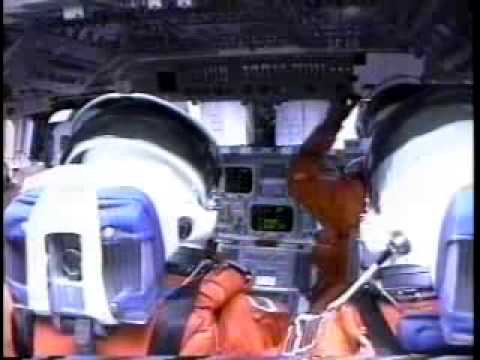The image depicts the slightly blurry interior of the Space Shuttle Columbia, taken from the rear of the astronaut seating area. The scene captures the launch cockpit view with three astronauts visible, all dressed in orange flight suits and white helmets. The pilot and co-pilot are seated side by side in the front, each strapped securely into blue headrest seats and facing forward, focusing on the complex array of control panels and instruments before them. The astronaut in the front appears to be adjusting a control on the dashboard with his left hand. The third astronaut is situated further back, also belted in, adding to the sense of preparation and activity within the shuttle. Despite the blurriness, the elaborate instrumentation and the intensity of the launch preparation are evident, conveying a powerful image of space exploration.